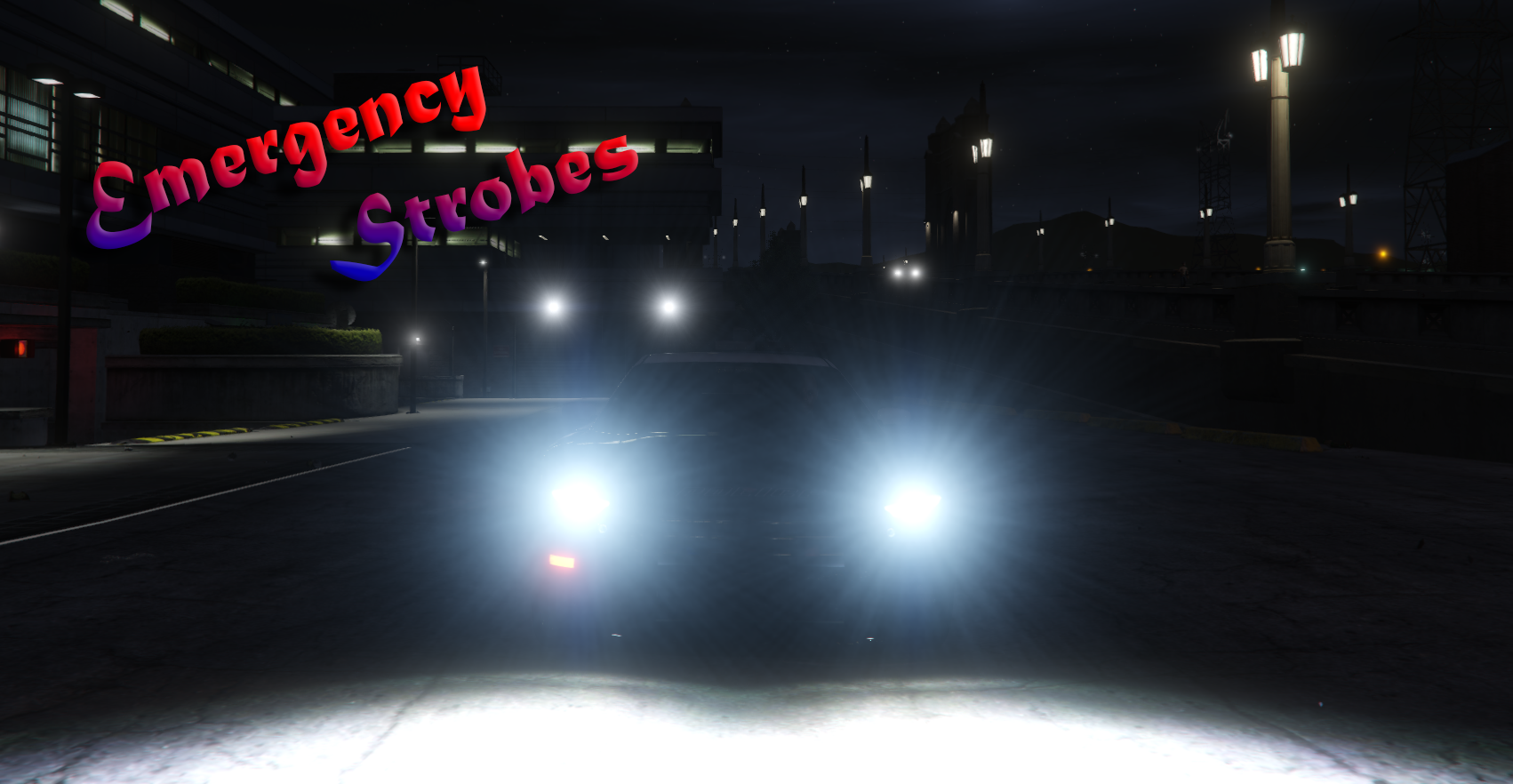In this drawing of a nighttime scene, we see the bright, blue-tinted LED headlights of an approaching car, shining forward and illuminating the ground directly in front with a stark white light. The car itself remains indistinct due to the intense glare of the headlights. The road below the lights reveals a few wrinkles and slits in the pavement. In the background, on the upper right side, there is a light gray pole with two conical streetlights, and additional similar light poles recede into the distance. To the left of the image, silhouetted buildings loom, and near them stands a person with a small white light illuminating them. Further in the background, more white lights suggest the presence of another vehicle. The sky above is a gradient of dark gray and black, signaling the night. In the upper left corner of the image, the words "EMERGENCY STROBES" are written diagonally and tilted to the left in a font that transitions from blue at the top to red at the bottom, adding an urgent, illuminated effect to the scene.